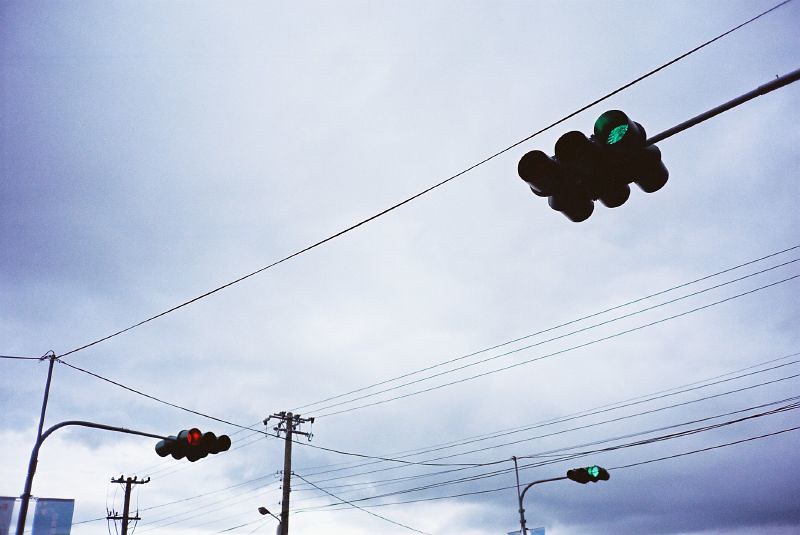The photo captures a striking scene shot directly into a notably cloudy sky, suggesting imminent rain. Dominating the image are numerous power poles and roughly a dozen power lines stretching horizontally from one side to the other. Prominently featured are three uniquely designed black traffic lights, each with lights arranged horizontally. The two traffic lights facing the camera display green signals, while the one facing away shows red. Notably, there are blue-colored banners hanging from the power line near the red light. Additionally, a streetlight extends from one of the poles, likely for nighttime visibility, enhancing the functionality of this intricate web of urban infrastructure.